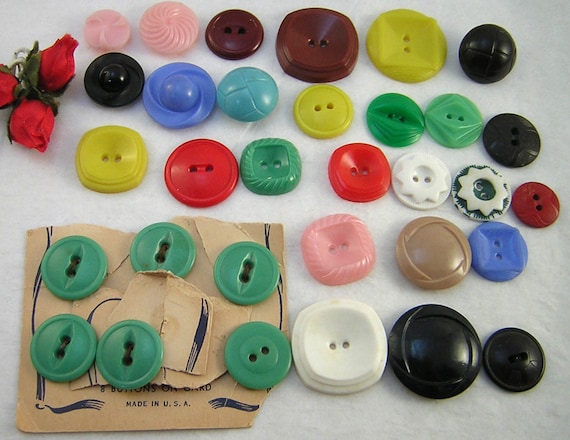This photograph captures a diverse assortment of 32 buttons in various colors, shapes, and sizes artistically spread out over a marble-like surface. Most buttons feature two small holes for threading. In the top left corner, there is a charming cluster of three small fabric roses. Below these, a series of nine buttons spans vertically, moving from pink to pink, brown, black, blue, blue, yellow, red, and green. The bottom left corner holds six turquoise buttons resting on a piece of paper or perhaps packaging that reads "Made in USA," adorned with decorative edges and possibly stating "eight buttons." More buttons in black, brown, blue, pink, and white are located on the bottom right side of the image. The top right displays twelve marbled buttons in a color sequence of brown, yellow, black, yellow, green, green, black, red, white, and a star-shaped blue button, capped with a dark maroon one. This striking collection rests on an elegant white-grayish background, perfect for crafting.